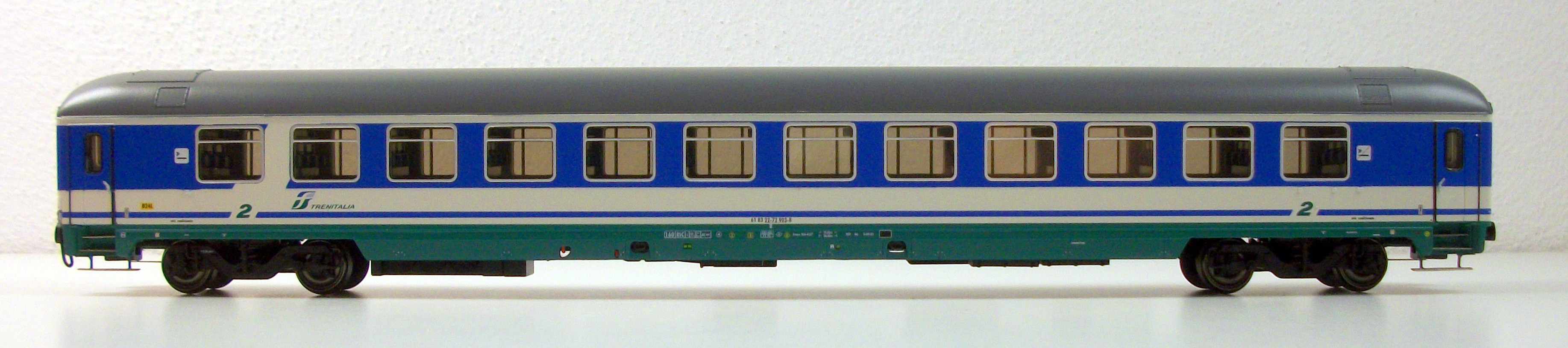This close-up, side-view photograph depicts a detailed model of a blue and white passenger train car placed on a white countertop, casting a shadow. The train car features a gray, rounded roof and a distinct color pattern along its body: a greenish-blue line just above the wheels, followed by a thin white stripe, then a wider blue stripe that runs through a row of approximately a dozen windows with white frames. Below the blue, there's another white stripe with a thin blue line underneath it. The train is equipped with a set of four black wheels at both the front and rear, though only two are visible at each end from this angle. There are small doors positioned towards the front and back, each accompanied by little step-up ladders. The carriage ends have numbered '2' markings, and there are green tubes positioned at both the front and rear ends of the carriage.